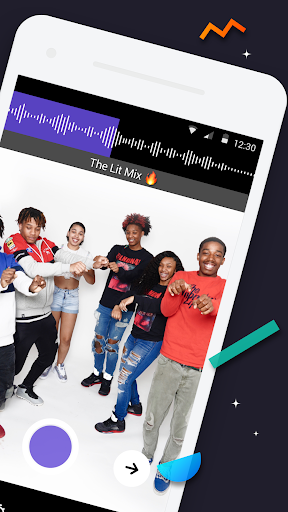The image features a complex design set against a black background. Central to the design is a large, stylized "M" in vibrant orange and red hues, accompanied by several four-pointed stars. A green bar and a blue half-moon add additional elements of color and shape. Overlapping this background, a white electronic device—possibly a cell phone or tablet—displays an image of six young people, all of whom appear to be teenagers or in their early twenties. They are dressed casually in jeans, T-shirts, and long-sleeve shirts, and their silhouettes are rendered in black.

Overlaying this group image is a graphic of sound waves in white, accompanied by the text "The Lit Mix" written in white font on a gray band. The left side of the image features a purple background, while the sound waves themselves are set against a black background. Below this central arrangement, a prominent purple circle appears, which may be a design element or a magnification button. Additionally, there's a white circle with a black right-arrow icon. The overall color scheme of the image includes blue, red, brown, white, purple, and green.